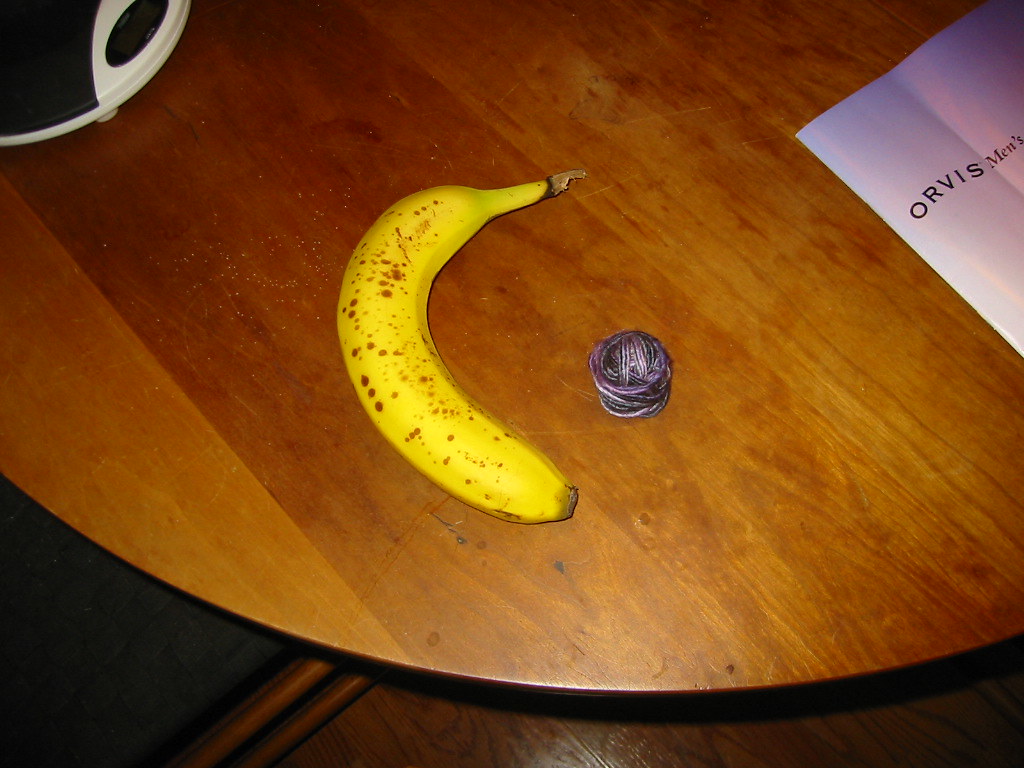In this photograph taken in Andorra, a ripe yellow banana with brown spots sits prominently in the center of a wooden table. To the left of the banana, there is a blue ball of twine that transitions to a reddish hue. On the far right side of the table, a white owner's manual with the word "Orvis" printed in black letters is clearly visible. Additionally, in the upper left corner, there is a white trivet or potholder with a black base. Behind the table, a chair with a gray cushion and brown legs can be seen, and the scene is set against a backdrop of a hardwood floor.